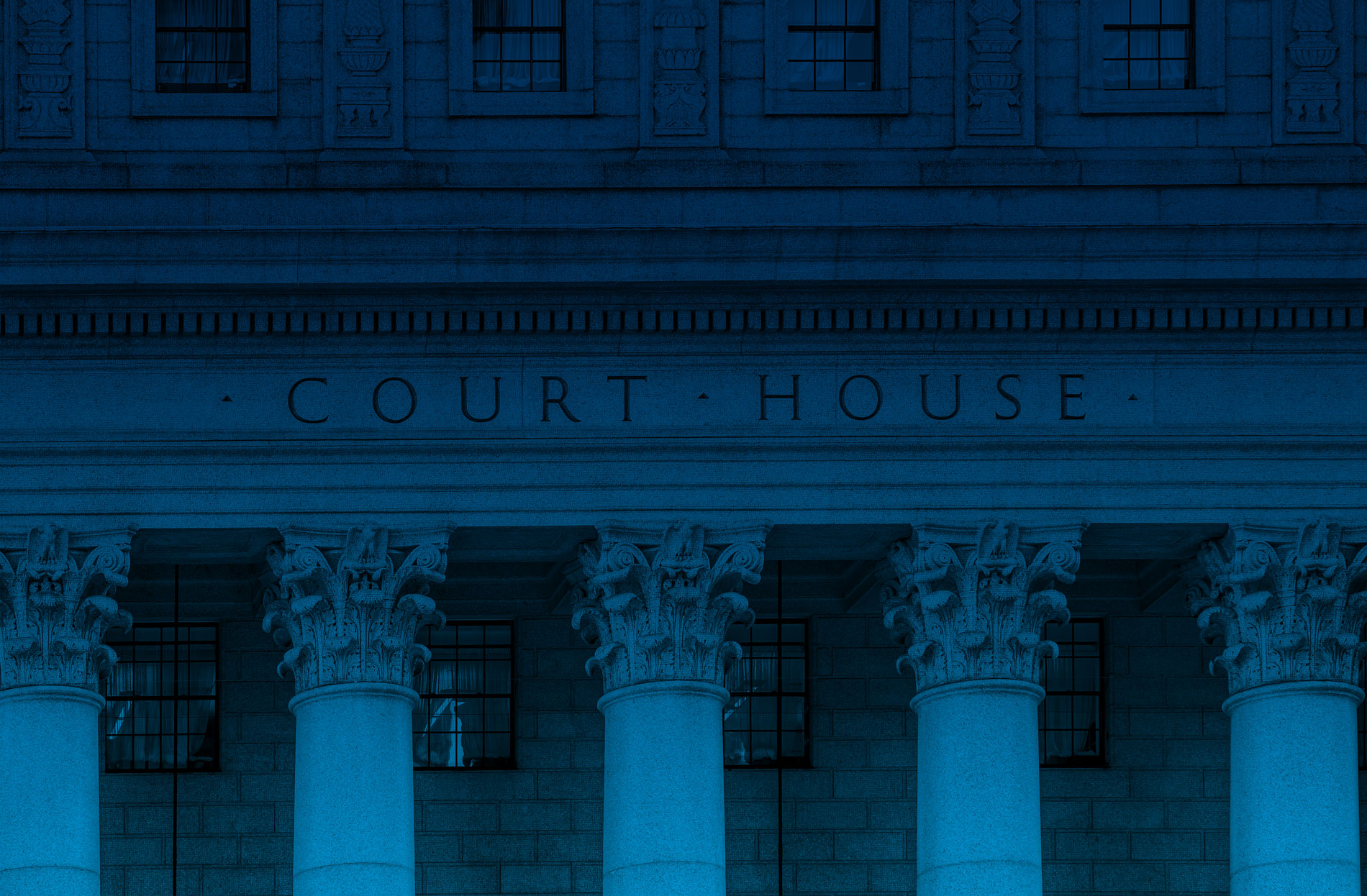The image is a dark-tinted color photograph of a large, classical courthouse building, captured in landscape orientation. The building, constructed from white or gray stone, exudes an imposing presence. The photograph highlights the entrance of the courthouse, focusing on five tall round columns that support an overhead structure. Each column features ionic flourishes, adding a touch of classical elegance. Centered above the columns, a black sign reads "Courthouse." The building's façade reveals four rectangular windows at the top, divided into small squares by intersecting lines. The photograph appears very dark, possibly due to the time of day or the camera's lens, with the entire image exhibiting a blue-tinted effect.